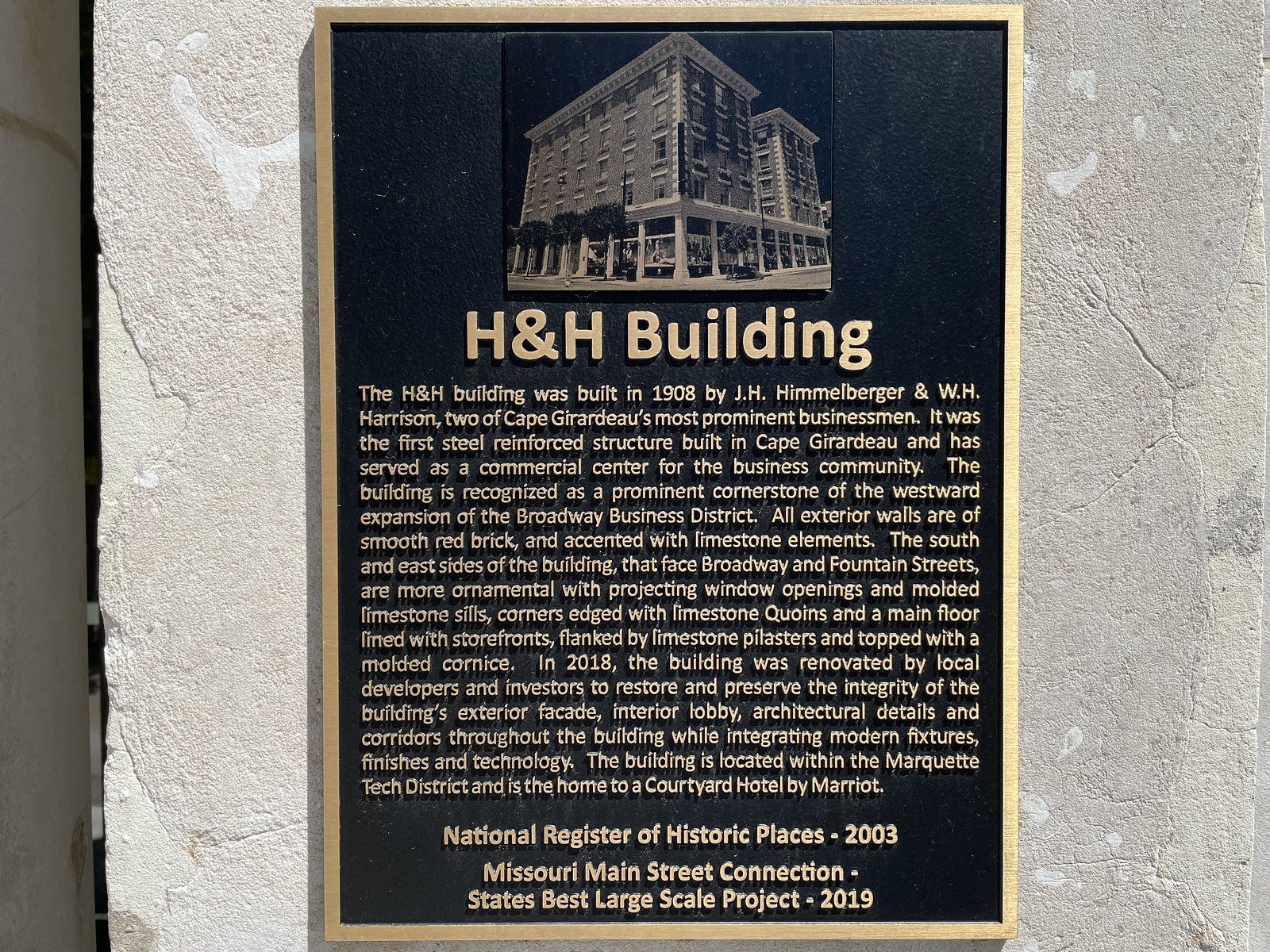This detailed description combines the key elements from the three given captions to form a cohesive and comprehensive caption:

---

The image shows a large, ornate plaque set against a cement backdrop. The plaque is black with gold borders and lettering. At the top, there is an etched depiction of an old building. Beneath this image, bold letters read "H&H Building." The plaque provides a detailed history, stating that the H&H Building was constructed in 1908 by J. H. Himmelberger and W. H. Harrison, who were notable businessmen in Cape Girardeau. This building was the first steel-reinforced structure in the city and has long served as a commercial hub, marking a significant part of the Broadway Business District's westward expansion. The structure features smooth red brick walls and limestone accents, with the south and east sides, which face Broadway and Fountain Streets, being particularly ornate. These sides include projecting window openings, molded limestone sills, quoined corners, and a ground floor lined with storefronts flanked by limestone pilasters and topped with a molded cornice.

In 2018, the building underwent a renovation to preserve its historic exterior facade, interior lobby, and architectural details while incorporating modern features. Located within the Marquette Tech District, it now houses a Courtyard by Marriott hotel. Near the bottom of the plaque, raised gold letters note that the building was added to the National Register of Historic Places in 2003 and received Missouri Main Street Connection’s State's Best Large Scale Project award in 2019.

---